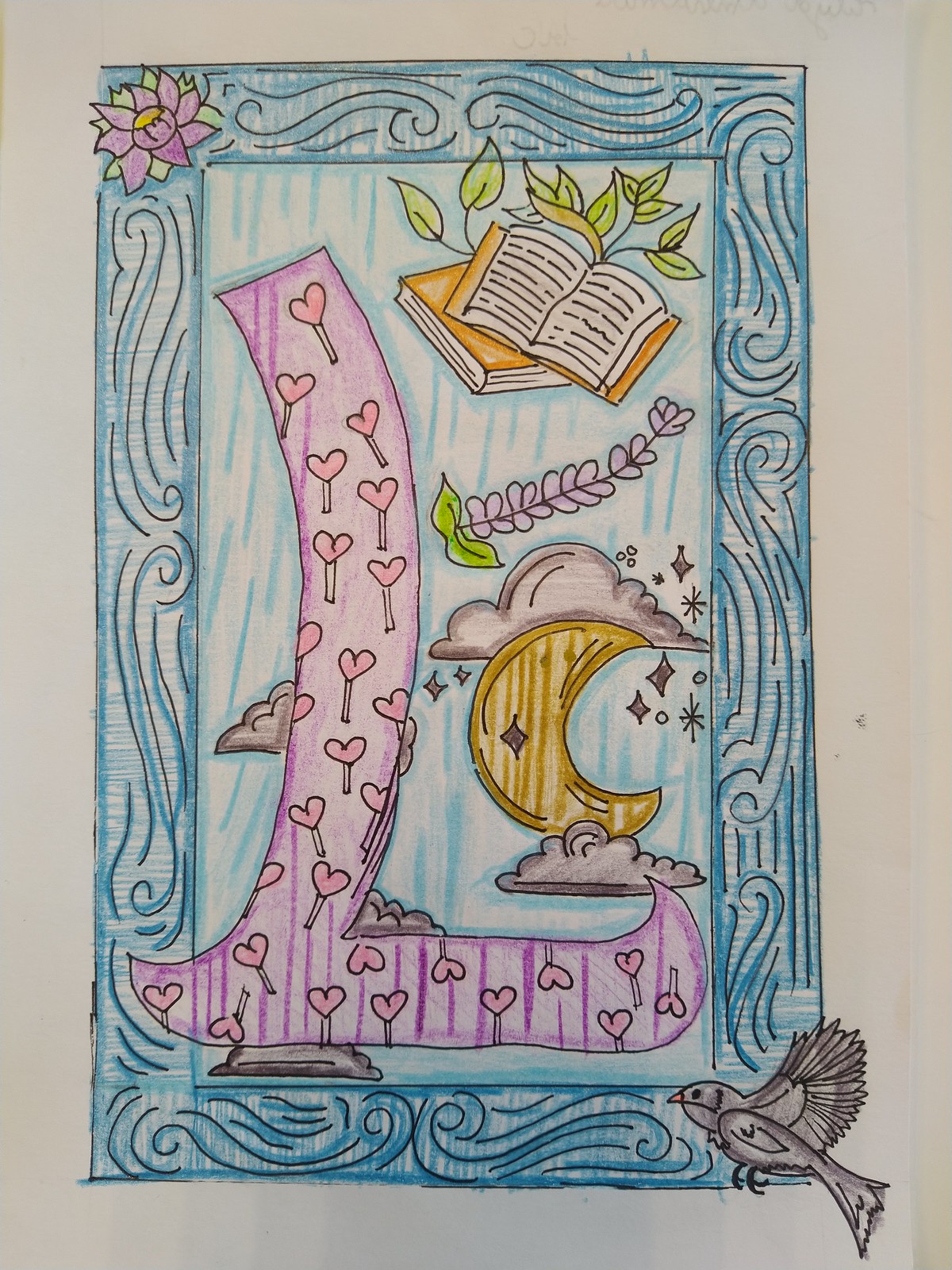A beautifully colored page features a rectangular artwork set against a gray background. The artwork is framed by a thick, blue-colored border adorned with intricate scalloped designs. In the lower right-hand corner, a gray bird perches partially on the artwork, with its tail and part of its wing extending onto the background. The upper left corner showcases a vibrant pink flower with a yellow center, surrounded by green leaves.

Dominating the center of the image is a light blue background. In the top left corner of this blue section, two orange books sit stacked, one open on top of the other, with green leaves sprouting above them. Beneath the books, a single long-stemmed flower with adjacent leaves adds a touch of elegance. Further down, a whimsical cloud floats, cradling a crescent moon colored in enchanting shades of orange and brown, and another cloud rests below it.

To the left side of the image, a large, wide letter "L" stretches vertically, painted in a soft pink hue. This "L" is embellished with pink hearts, each suspended from delicate black-outlined stems, contributing to the overall charm. The hearts are slightly different in shade from the "L," creating a harmonious yet varied color palette.